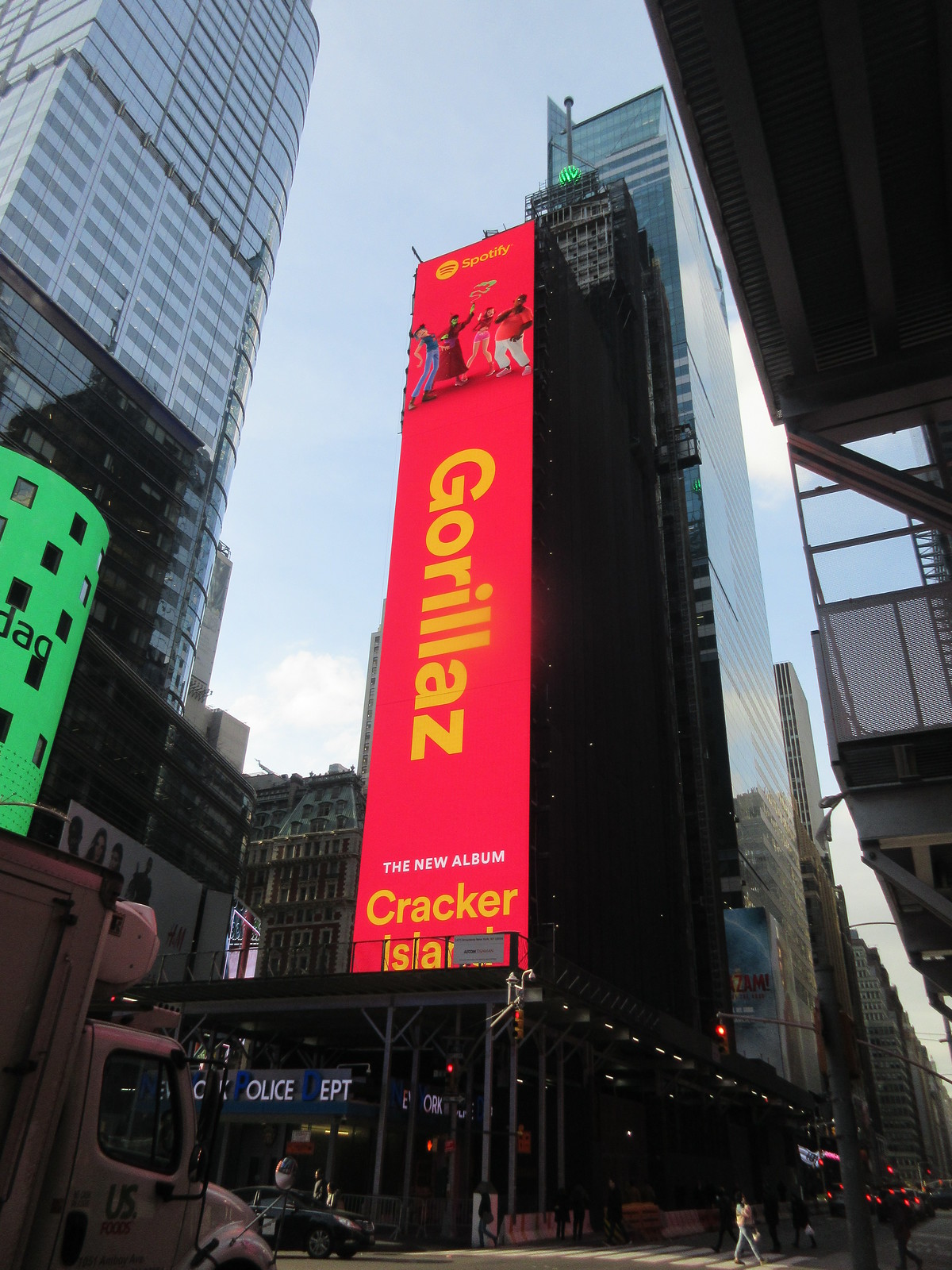A vibrant daytime photograph captures a bustling cityscape from street level, reminiscent of a scene in New York City. Dominating the center is a towering, older skyscraper with a massive digital billboard that stretches vertically up the building, shining a striking red hue. This billboard prominently advertises the Gorillaz’s new album "Cracker Island" with yellow lettering. At the very top, the Spotify logo indicates it's an ad. The billboard also features faint images of four dancing figures. Additional modern glass skyscrapers frame the primary building, extending out of the frame, with one slightly to the left. Street-level activity includes a partially visible box truck with an air conditioning unit and a solitary figure walking across the street. In the lower portion of the frame, an obscured sign suggests the presence of a police department, hinting at a bustling urban environment rife with detail and energy.